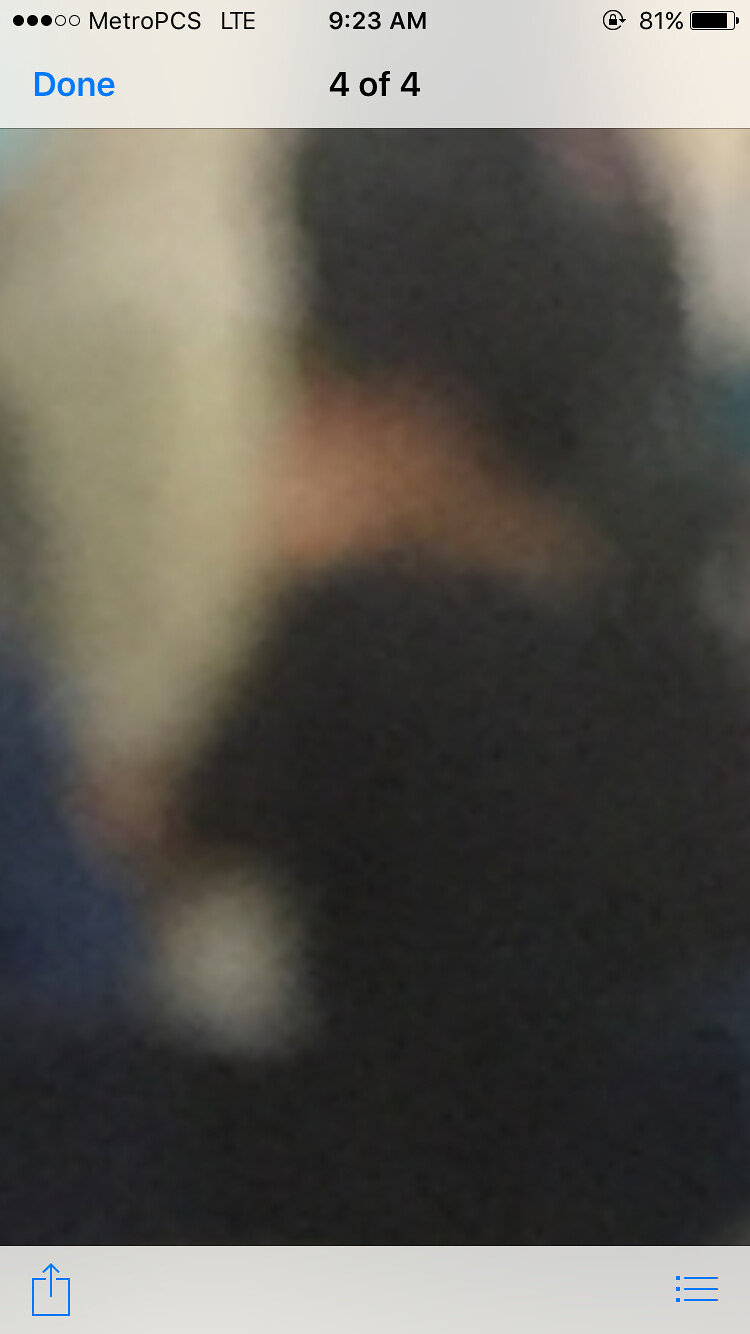The image displayed on a cell phone screen shows a blurred and dark photograph, possibly of a person with long hair wearing a black shirt, looking away. The top of the image features a white strip with several indicators: five circles at the top left, three filled in black and two unfilled, followed by the text "Metro PCS" and "LTE." In the top center, the time is displayed as "9:23 AM," and on the top right, there is a lock icon next to "81%" with a nearly full battery symbol shaded in black. Directly below the white strip, the text "Done" appears in blue at the top left, and "4 of 4" is centered in black. The bottom of the image has another thin white strip; on the left is a blue square with an upward arrow, and on the right, three blue horizontal lines with three dots in front. The blurred image appears to mostly consist of dark colors, with some areas of blue and white blobs, and a hint of purple in the bottom left corner.